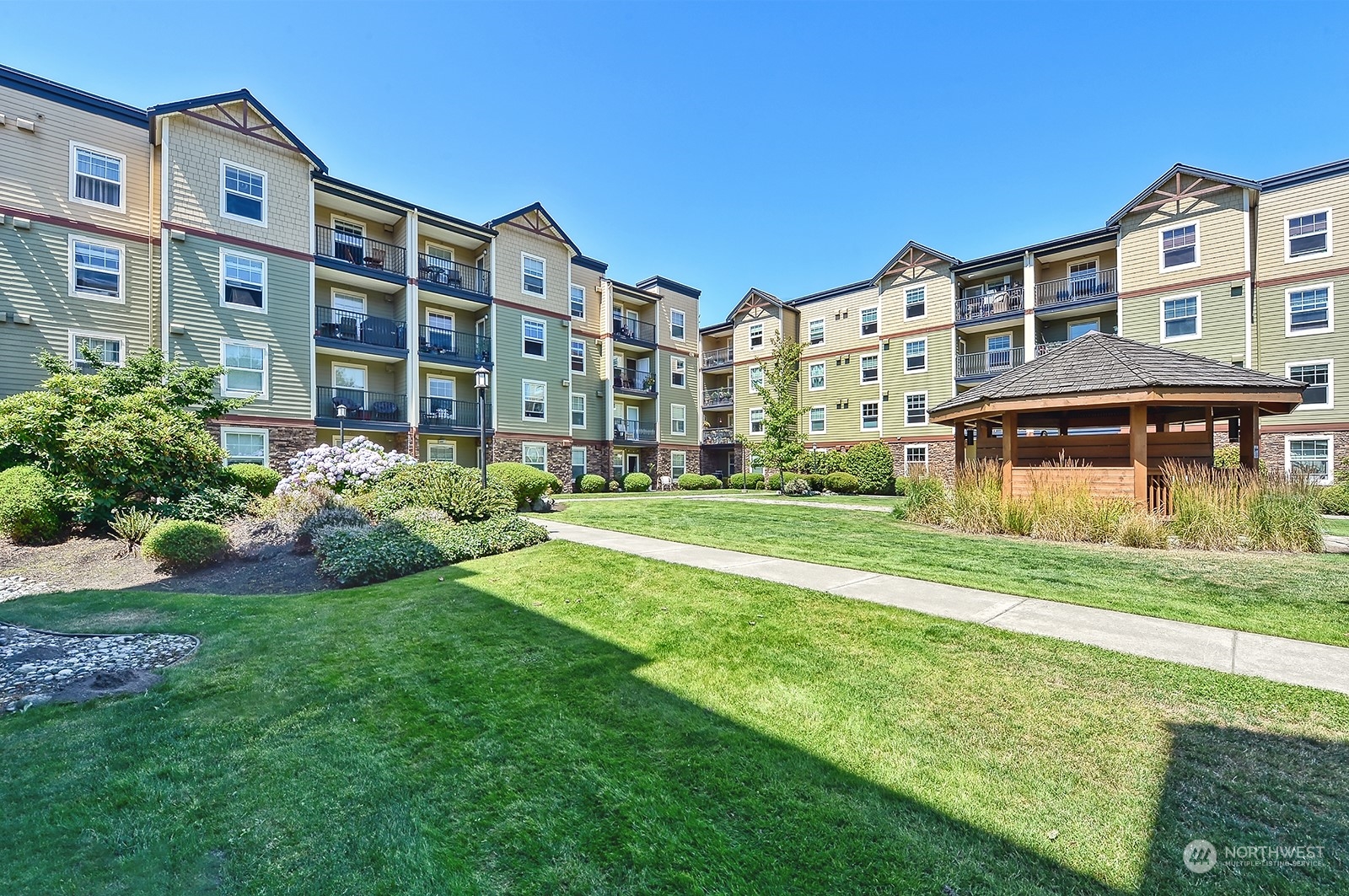The image depicts a meticulously maintained courtyard in front of a four-story apartment complex. The buildings, seen at a perpendicular angle, are multicolored with a top layer of yellow or tan, middle layers of green, and a ground floor of brick. Each building features rows of evenly spaced windows, around thirty-two per building, and various decks adorned with outdoor furniture. The expansive grassy area is complemented by well-tended shrubs and evergreens, particularly concentrated on the left side. On the right side stands a wooden gazebo or pergola, surrounded by tall grasses and bushes, providing shade and an inviting spot to relax. The sunny day casts shadows across the lush lawn, with a diagonal sidewalk running from the lower right to the center of the image, leading viewers through this serene recreational space. The only text in the image, located at the bottom-right corner, reads "Northwest."